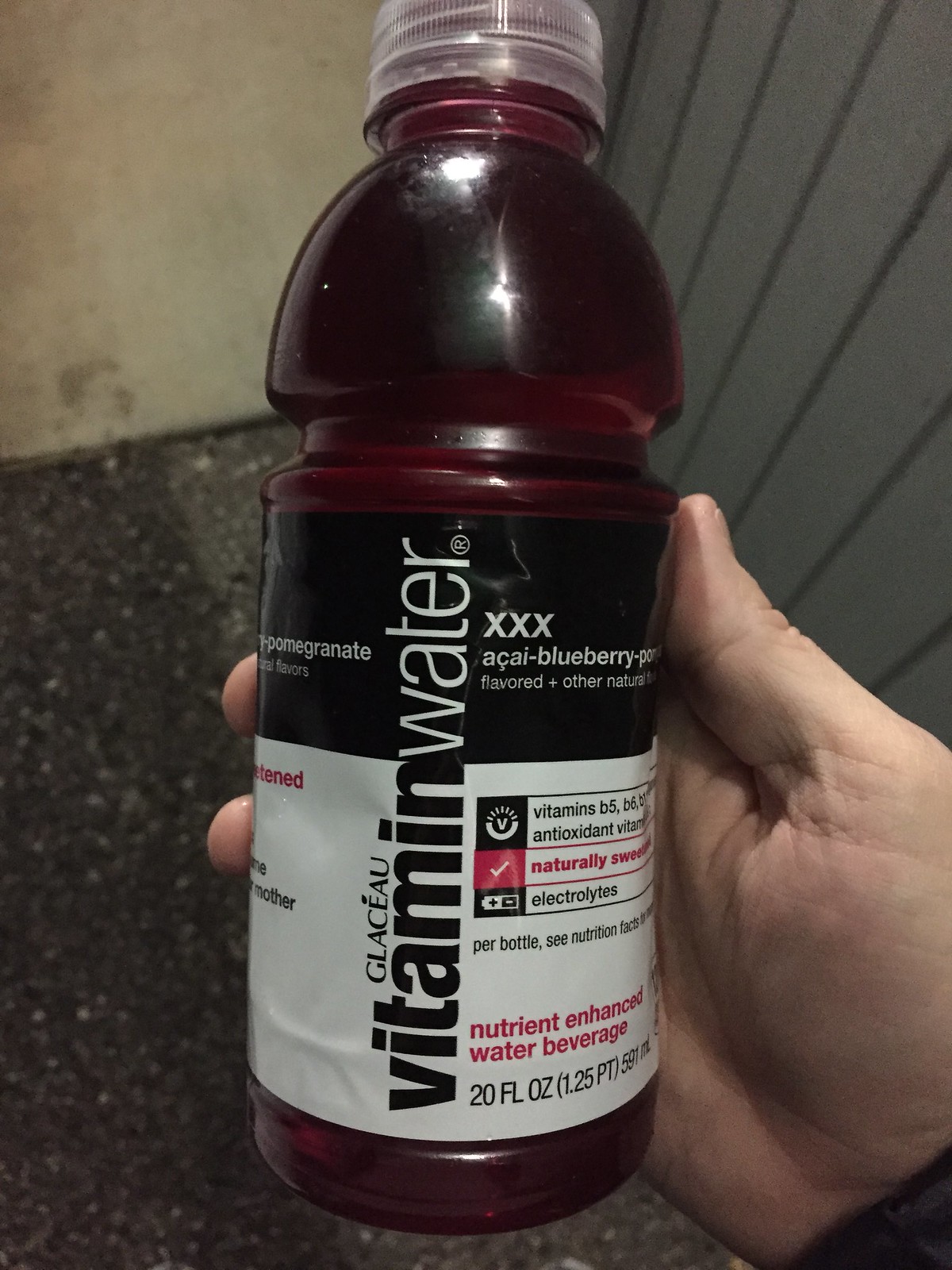In this photograph, a person holds a bottle of Glaceau Vitamin Water up to the camera, prominently displaying the bottle's features. The beverage inside the clear bottle is a rich, dark burgundy color, contrasting with the transparent lid and the detailed label. The label itself is predominantly black and white, interspersed with sections of the same burgundy hue. On the label, the brand name "Glaceau Vitamin Water" is printed vertically, while the flavor, identified as acai-blueberry-pomegranate, is partially visible, with the letters "P-O" hinting at pomegranate.

The hand holding the bottle appears to belong to a white individual, identifiable by the visible thumb and portion of the hand. The person is wearing a dark shirt, of which only the sleeve is partially visible in the frame. The background adds texture to the image, featuring a dark spotted floor that resembles pavement, a stark white wall, and a section of gray siding composed of vertical slats. This detailed composition captures not only the beverage but also the context in which it is presented, providing a rich visual narrative.